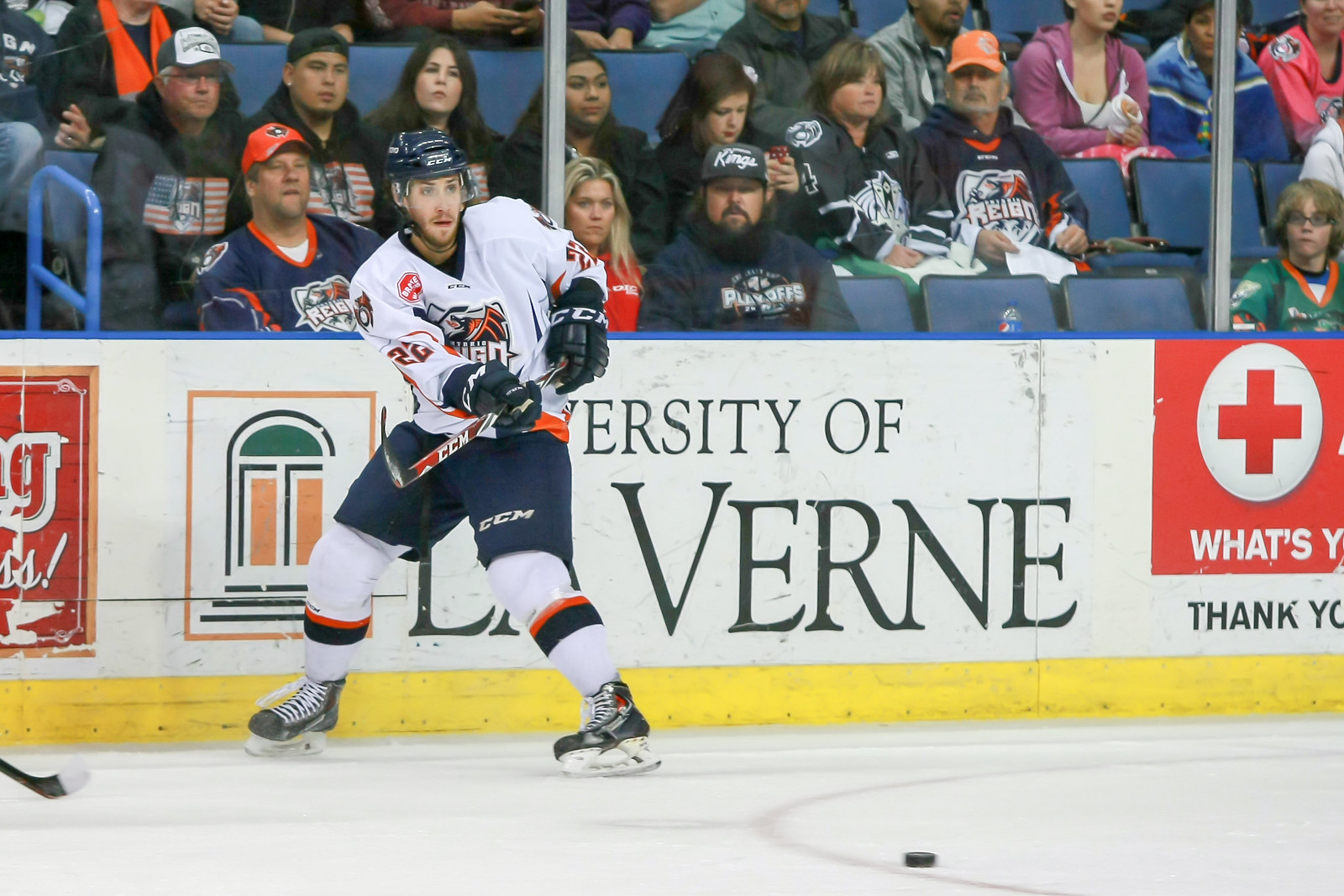This image captures a dynamic moment during a professional hockey game, highlighting a single player who is positioned slightly left of center. The player is dressed in a blue and white jersey with orange accents, blue shorts, a dark blue helmet, and black hockey gloves. His stick is raised, suggesting recent action with the puck, which is visible on the ice near the bottom, slightly right of center. 

In the background, behind the glass wall of the rink, approximately 15 spectators are seated. Notably, two individuals are wearing orange caps, and at least three others don jackets featuring an American flag logo. In the upper right corner of the stands, a person in a pink top can be seen, and two rows over, two seats to the right, someone is wearing a purple jacket.

The rink's boards display various advertisements, including a prominent one for the University of La Verne, with a partially readable "University of Laverne" sign in black letters. To the right of this, there is another ad featuring a Red Cross emblem and the fragmented text, "WHAT'S." Additionally, there is a phrase thanking donors, though the clarity is compromised as the U's are cut off. A yellow line runs along the bottom of the boards, completing the frame of the action shot. The main colors in the image are white, blue, and red, contributing to a vibrant and engaging scene.